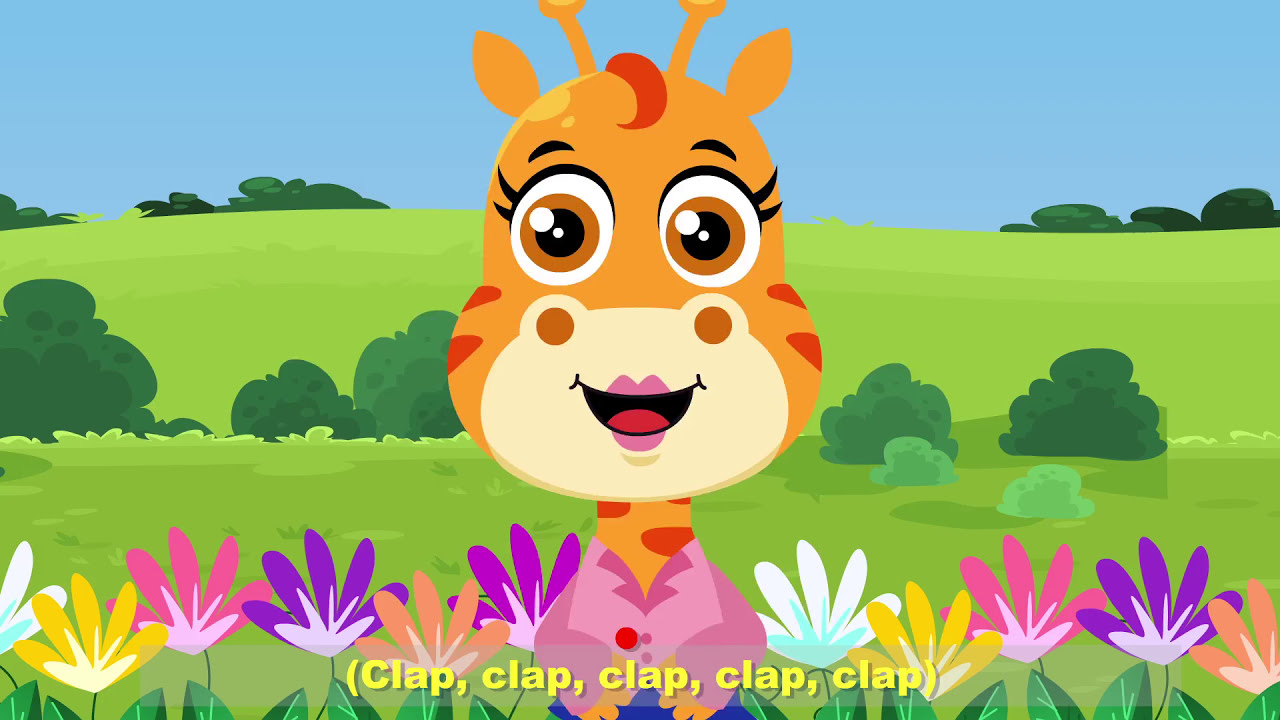The illustration shows a colorful cartoon scene set in a landscape format, dominated by a cheerful, cartoony giraffe at the center. The giraffe has a disproportionally large head with a tuft of red-orange curly hair and two antennae. Its face features big round gold eyes with black eyelashes, a smiling mouth with visible purple and pink lips, and a red tongue. The giraffe is dressed in a purple long-sleeved shirt and blue jeans.

The background includes a light blue sky giving way to rolling green meadows. A horizontal band of darker green bushes lines the middle of the scene, with scattered trees on both the left and right sides. There is a vibrant row of blooming flowers—white, yellow, pink, purple, and rose—that runs horizontally behind the giraffe. 

At the bottom of the image, yellow sans-serif text in parentheses reads "clap, clap, clap, clap, clap," with a bouncing red ball above the middle "clap," indicating a rhythmic clap-along for viewers. The scene is designed in a juvenile-friendly illustrative style.